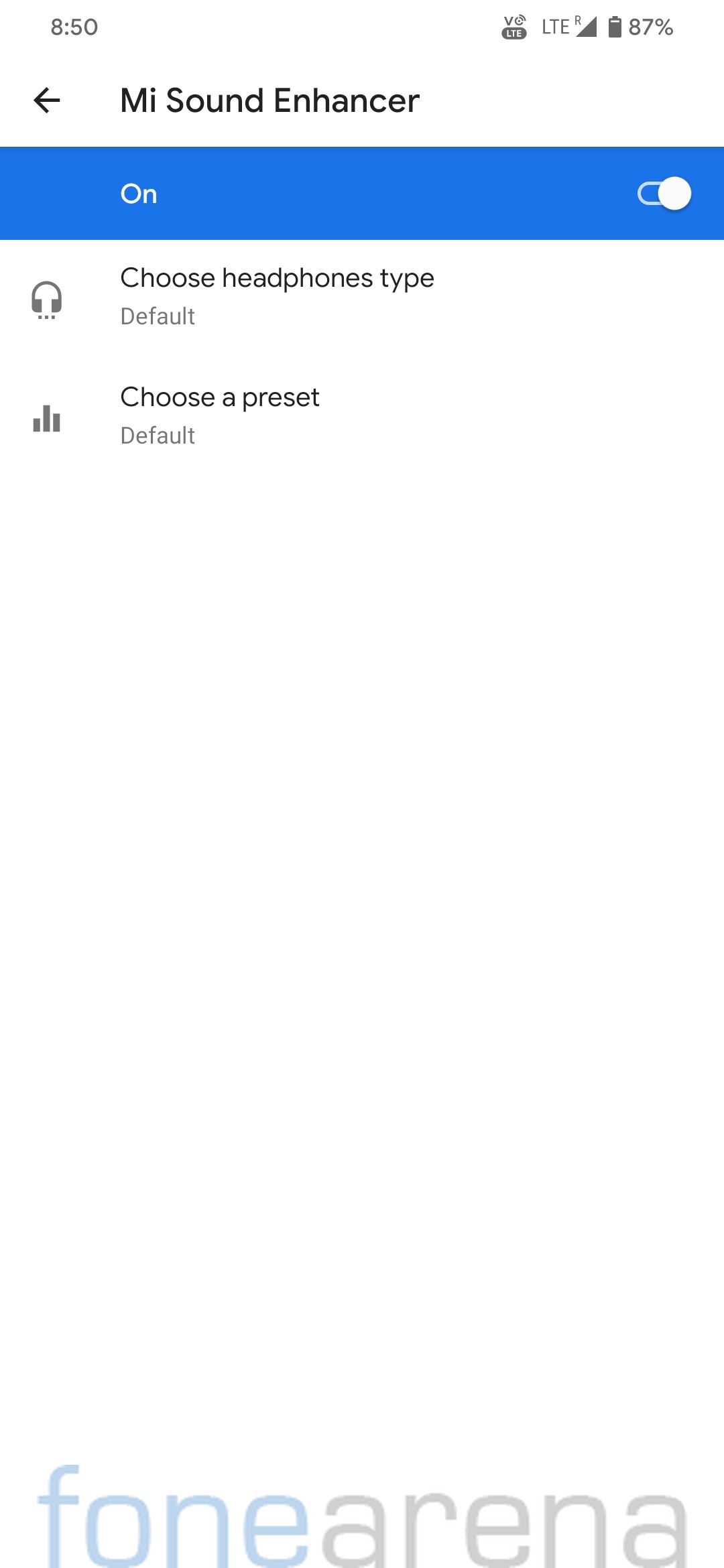The image is a vertically rectangular cell phone screenshot with an all-white background. The status bar at the top features "850" on the left, and multiple icons on the right, including LTE, signal strength, and a battery icon showing 87% charge. Below this, there's a headline reading "Mi Sound Enhancer" with a left-pointing arrow icon to its left. A horizontal blue banner underneath displays the word "ON" in white with a toggle switch on the far right. Further down, there's a headphone icon next to the text "Choose headphone type: Default". Below that, there's a bar icon with text "Choose a preset: Default". At the very bottom of the image, "Phone Arena" is written in light blue and gray.